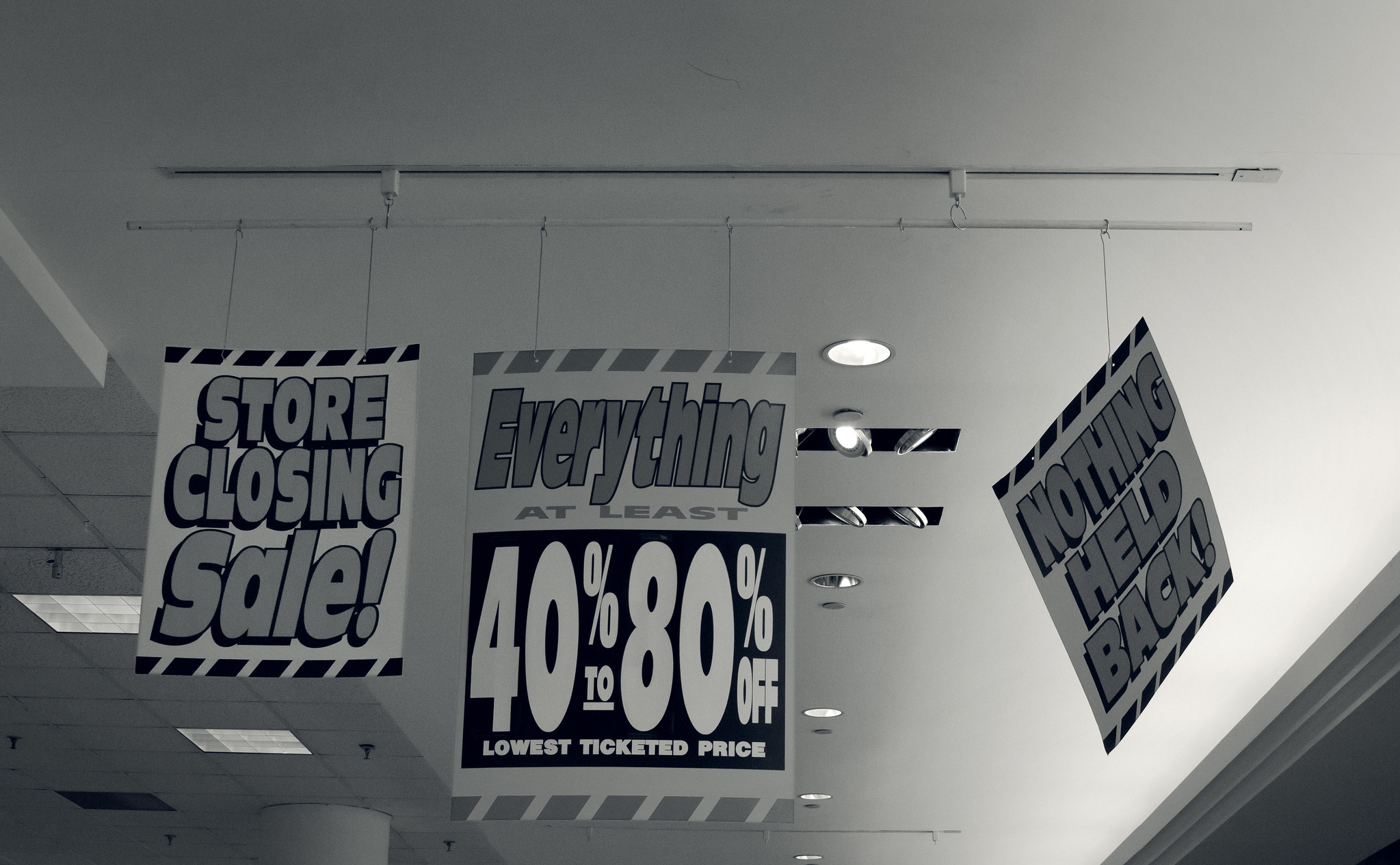This black and white photograph captures the interior of a retail store in its final days. Three prominent signs hang from the ceiling on a long rack, stretching from left to right, and convey the urgency of a store-closing sale. These signs are suspended by strings, enhancing the scene's sense of impermanence. 

The first and third signs are identical in design; they are white with black trim at the top and bottom, and feature bold, dark gray lettering outlined in black. The message on both reads "STORE CLOSING SALE!" The first sign is securely hung by two strings, while the third sign appears to have partially fallen, hanging precariously by a single string on its right side, as if the left string has come loose.

At the center, the largest sign draws immediate attention, positioned lower than the others. It boldly announces, "EVERYTHING AT LEAST 40% TO 80% OFF, LOWEST TICKETED PRICE," emphasizing the depth of the discounts. Like the other signs, it shares the same color scheme and is held up by two strings, ensuring its prominent placement.

Overall, the scene captures a moment of transition, filled with both the promise of bargains and an atmosphere of finality.